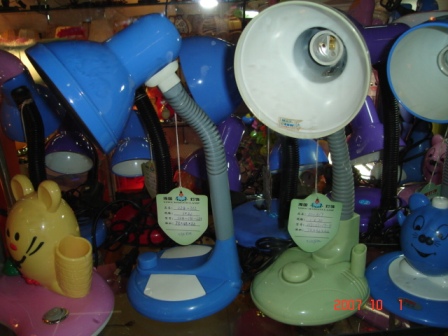This photograph depicts a collection of vibrant children's desk lamps displayed on a tabletop. The central focus features two prominently positioned lamps—one being a bright green and the other a light blue, with bendable necks and rounded, bowl-like bases. Both lamps have small, hood-shaped shades that fan out, and each has an on/off button located in the middle of their bases.

Adjacent to the green lamp on the right, there is a blue figurine resembling a bear. On the left side near the blue lamp, there appears to be a yellow or pink-based lamp adorned with a cartoonish character, likely a bunny or cat. In the background, numerous other lamps in shades of purple and blue are visible, adding to the colorful scene.

The image, although of poor quality and poorly lit, suggests a display likely taken in a retail setting, evident from the hanging price tags affixed to the lamps. A date and time stamp in the lower right corner indicates the photo was taken on January 10, 2007.